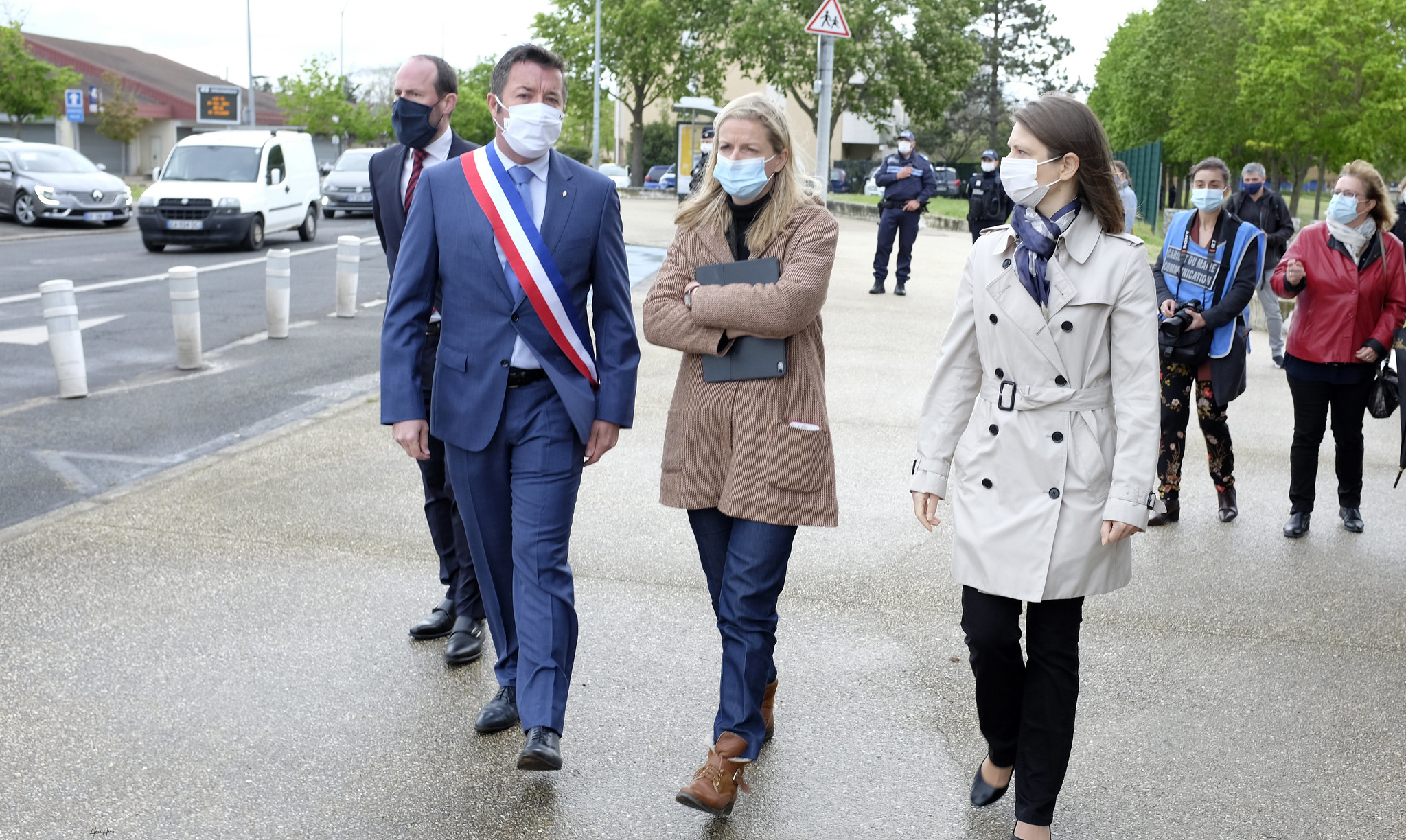A wide city sidewalk, approximately 20 feet in width, is bustling with people, all wearing face masks. Prominently, a man in a blue suit, white dress shirt, and blue tie walks with a tricolor blue, white, and red sash draped from his right shoulder to his left hip, reminiscent of the French flag. He appears to be around 40 years old. To his right, two women engage in conversation with him. The woman on the far right has brown hair and wears a white overcoat with black buttons, a scarf around her neck, black pants, and is looking towards the middle woman. The middle woman, who is blonde, is dressed in a brown sweater, blue jeans, and brown boots, and carries a black folder held close to her chest. To the left of the man in the blue suit, another man in a black suit with a burgundy tie and matching black face mask walks slightly behind. The sidewalk is adjacent to a road with visible white barricades cemented into the ground. Cars, including a white van and two four-door sedans, drive by while distant security personnel, reporters with cameras, and other pedestrians add to the commotion in the background.